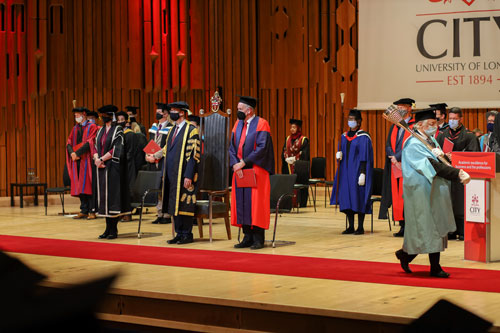This detailed color photograph captures a graduation ceremony on a small, beige wooden stage adorned with a modern, orange backdrop that features unique bamboo-like shapes with oval patterns. The stage has a red runner carpet crossing the front, where a person in an aqua robe can be seen walking off to the right side, holding an award. To the left and center, several dignitaries and professors stand in front of a large chair, wearing graduation robes, neck scarves, black face masks, and black hats, indicating the event took place during COVID-19. Behind them, other individuals in various colored long gowns and graduation robes are also present. A partially visible banner in the top right corner reads "University of London, established 1894," with another flag, slightly obscured, showing the word "City." The composition and attire suggest the formal occasion is held at the University of London.